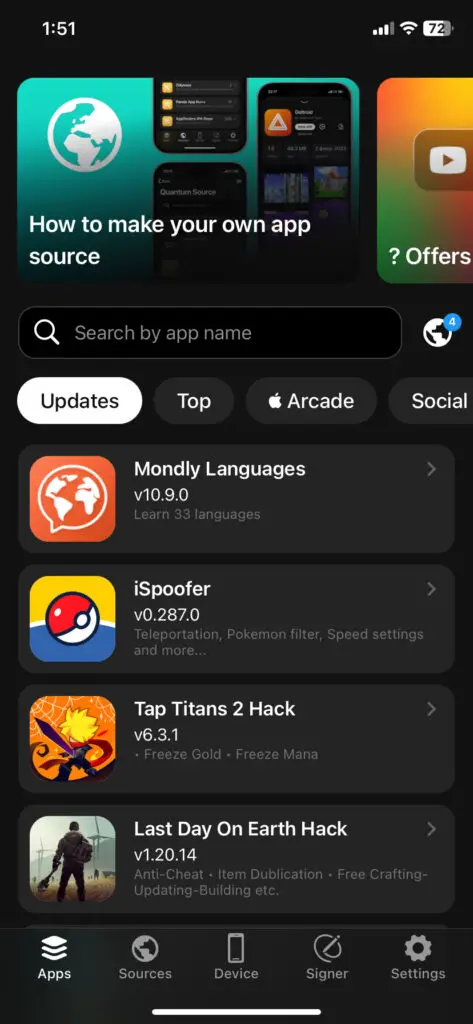This image is a screenshot of an app store-like interface taken from an iPhone. At the bottom of the screen, five icons are displayed from left to right: "Apps," "Sources," "Device," "Signer," and "Settings." Directly above this toolbar are four different apps listed vertically. 

- The first app, "Mondly Languages," has an orange app icon featuring a chat symbol with an earth inside it. It is identified as version 10.9.0, and the description highlights the ability to learn 33 languages.
- The second app, "iSpoofer," has a yellow and blue icon with a Pokémon symbol in the center.
- The third app is "Tap Titans 2 Hack," featuring an app icon with a small character wielding a sword.
- The fourth app, "Last Day on Earth Hack," displays an icon of a main character holding a weapon, standing in a field-like setting.

At the very top of this app list, there are three tabs labeled "Updates," "Top," "Arcade," and "Social." Above these tabs, there is a search bar that reads "Search by app name." Further above this bar is a small window that provides the option "How to make your own app source."

The entire background of the interface is black. In the status bar at the top of the screen, the time displayed is 1:51, and the battery percentage on the top right is shown to be 72%.